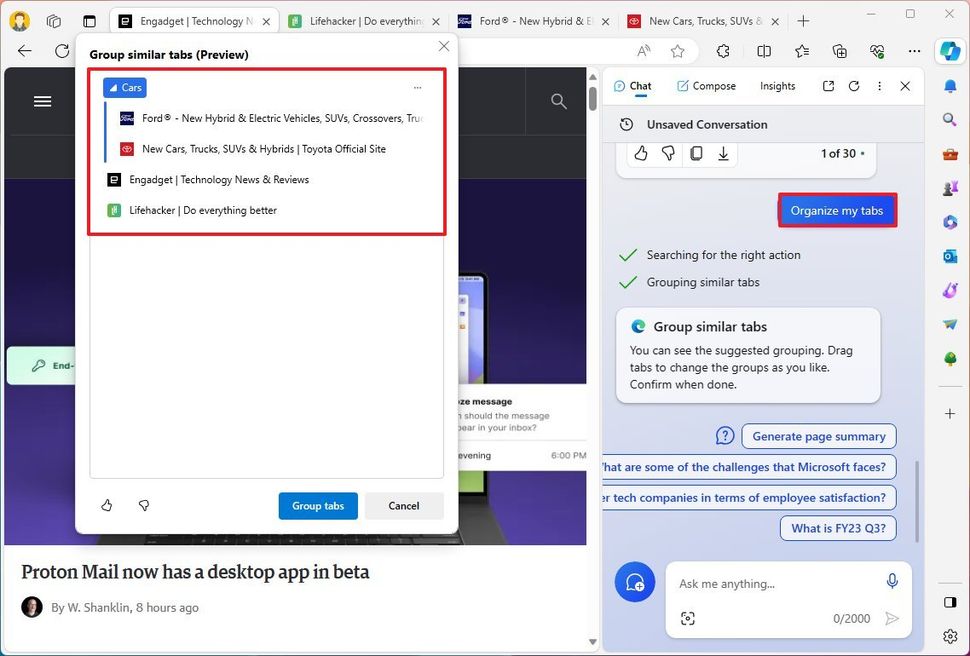This image captures a detailed screen of a website displaying various browser elements and a chatbot interface. 

At the top of the screen, there's a gray browser bar featuring standard icons and open tabs. These tabs include Lifehacker, Ford, and another with a red icon titled "New Cars, Trucks, and SUVs". On the far right of the browser bar, typical icons are visible: a circle with wavy lines, a book, a star, a square with a plus sign, and a profile icon, possibly representing the Google Copilot button. Further down the right-hand side, on a gray background, additional icons appear, such as a notification bell, a magnifying glass, a shopping cart, along with icons resembling chess pieces, a camera, and two green symbols.

To the left, a gray box prominently displays a section with an underlined "Chat" header. A white bar on top of this section reads "Compose" and "Insights", flanked by reload and X buttons. Within the gray background, there's a message stating "Unsafe Conversation" above a blue bar with white text that reads "Organize Tabs." This section includes elements like green check marks and phrases such as "Searching for the Right Action" and "Grouping Similar Tabs," suggesting it is a chat assistant helping to organize the user's tabs.

On the left side of the screen, a large vertical white text box is labeled "Group Similar Tabs Preview" in bold black text. The top right of this box features a gray X, and inside, there are bolded lines of text outlined in red. At the top left, a blue button labeled "Cars" appears, followed by organized text listings such as Ford, New Cars, Gadget Technology, and Lifehacker, matching the browser's open tabs. At the bottom, a blue bar with white text offers an option to "Group Tabs," while a white bar with black text provides a "Cancel" button.

The screen's sides have a purple background, and at the very bottom, a bold black text banner announces "ProtonMail now has a desktop app in beta." Next to this message is a profile icon and, to the right, the attribution "by W. Shacklin eight hours ago."